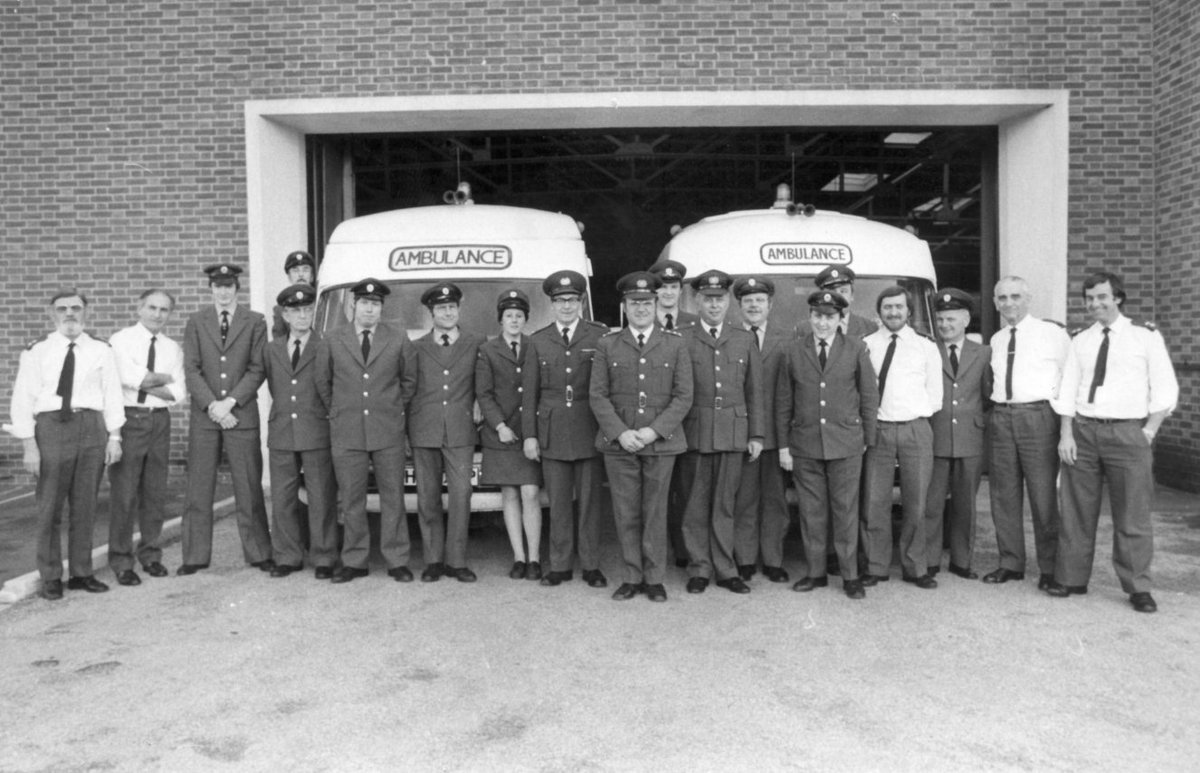In this black-and-white photograph taken in front of a red brick building, a group of approximately two dozen ambulance workers from the 1960s or 70s stands solemnly before two ambulances. The ambulances, taller than the people and emblazoned with the word "ambulance" in dark writing on their white upper sections, are parked outside a large garage door, which is open, revealing the spacious interior. The majority of the workers are dressed in uniform outfits consisting of dark jackets with gold buttons, long pants, ties, and hats adorned with small badges. They stand in orderly rows, with a few exceptions: about five individuals wear long-sleeved white shirts and ties instead of the full uniform, and there is one woman among the men, noticeable by her skirt. All are looking straight ahead, providing a sense of unity and formality in this historical snapshot of an ambulance crew.